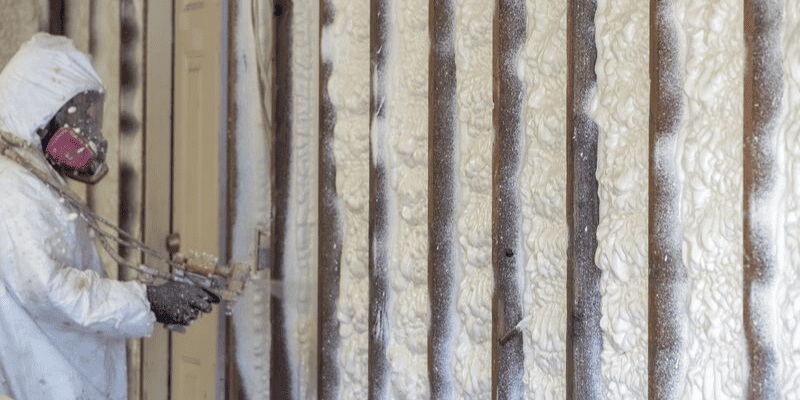In this detailed image, a person stands to the left, clad in what appears to be a white hazmat suit. They wear protective gear, including a pink air filter mask and black gloves. In their hand, they hold a metal sprayer, which they are using to apply white spray foam insulation onto the visible framework of a wall. The wall consists of vertical brown 2x4 wooden studs, preparing the structure for future drywall installation. Around their neck, brown ropes or straps are evident. To the left of the individual is a light yellow door framed in off-white. Behind them, additional sections of the wall have already been sprayed with foam, which transitions from white to an off-white or light yellow hue as it dries.